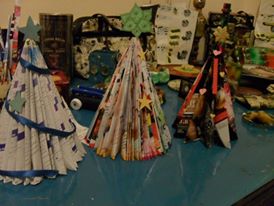This image features a scene on a dark blue, reflective, and shiny tabletop. At the forefront, there are three crafted Christmas trees, seemingly made from folded paper or cloth. Each tree boasts unique decorations: The tree on the left is white with blue squares and is adorned with a light blue star and a blue sash wrapping around it. The middle tree features a green star with a floral design, and its body is decorated in orange, white, and yellow hues. The right tree is black with a gold star on top and red lines cascading down it. In the background, the setting appears cluttered, possibly indicating a classroom, thrift store, or craft store. Visible are a wooden toy car with white tires, some Legos, and various other items. Bright overhead lighting illuminates the scene.